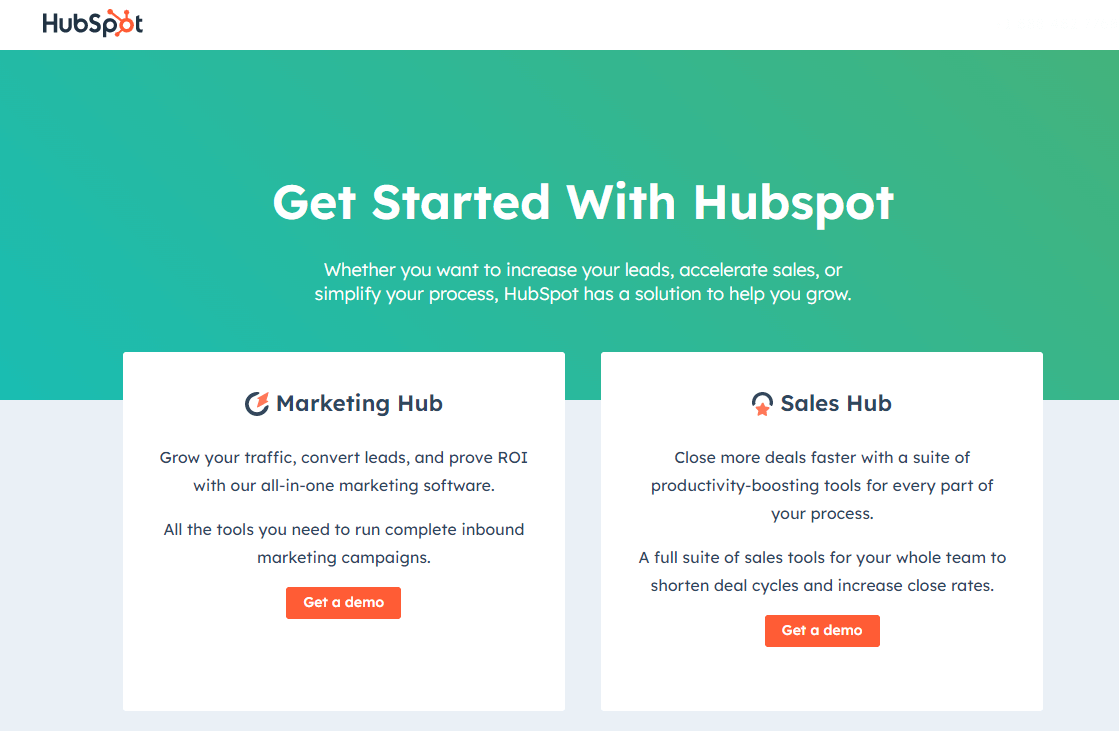This image is a screenshot of the HubSpot website, featuring a visually striking background with a gradient transition from teal on the left to bright green on the right. The lower portion of the image is light grey. In the upper left corner, the HubSpot logo is prominently displayed, with the 'O' stylized as a splash. 

Within the green gradient section, there is white text that reads: "Get started with HubSpot. Whether you want to increase your leads, accelerate sales, or simplify your process, HubSpot has a solution to help you grow." 

Below this text, two white rectangular blocks are partially set against the green and light grey sections. The left block is labeled "Marketing Hub" and includes the tagline, "Grow your traffic, convert leads, and prove ROI with our all-in-one marketing software. All the tools you need to run complete inbound marketing campaigns." Beneath this description is an orange button with white text that says "Get a Demo."

The right block is labeled "Sales Hub" and features the message, "Close more deals faster with a suite of productivity-boosting tools for every part of your process. A full suite of sales tools for your whole team to shorten deal cycles and increase close rates." An orange button below this text also reads "Get a Demo."

Overall, the screenshot effectively conveys HubSpot's offerings for both marketing and sales tools, emphasizing their capability to enhance business growth and efficiency.